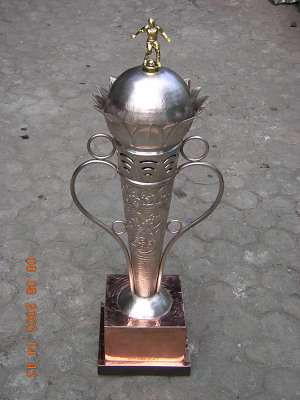The image is a rectangular photograph, likely taken outdoors in natural lighting, from a standing perspective looking down at the ground, which is covered in gray, interlocking stone. The central focus of the photo is a trophy placed on this brick ground. The trophy has a copper-colored, square base that supports a silver, cone-shaped body. Adorning the sides of the silver cone are handles that form heart-like shapes, possibly serving as handgrips. The upper part of the trophy transitions into a circular form topped with a small gold figure of a soccer player posed as if kicking a soccer ball. This suggests that the trophy is awarded for soccer achievements. The image also features a blurry orange date and time stamp in the left-hand corner and possibly some unreadable text on what appears to be a white table or platform beside the trophy.